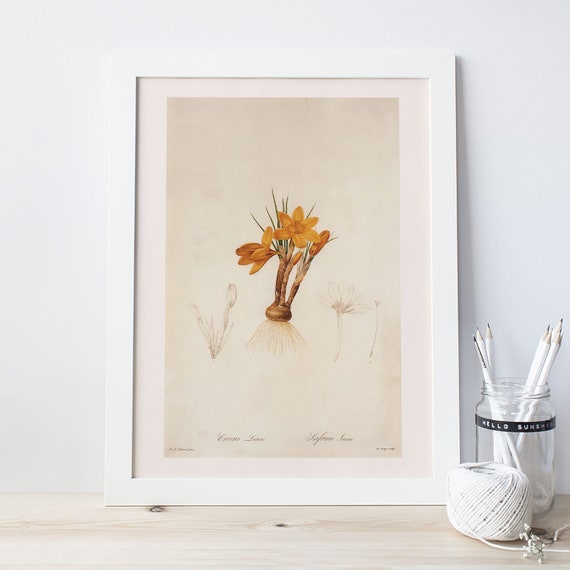The image features a serene, minimalist setup anchored by a botanical painting at the center. The painting is encased in a white frame, with a matching white mat, and it depicts several orange flowers with dark green leaves and visible roots, possibly from the lily family. The flowers are in various stages of bloom: the left stem shows a partially opened flower, the center stem boasts a fully opened yellow day lily, and the right stem bears a long, oblong yellow bud. Pencil sketches depicting preliminary designs of the flowers flank the main image, adding an artistic touch. Below the painting, there is an artist's signature written in black script, though it's too small to read.

To the right of the painting sits a clear glass canister with a black label that reads "Hello Sunshine," filled with white pencils, a white paintbrush, and a skein of white thread positioned in front of it. This setup rests on a light wooden surface that resembles whitewashed wood, all set against a plain white wall. The combined elements create a crisp, artistic ambiance.